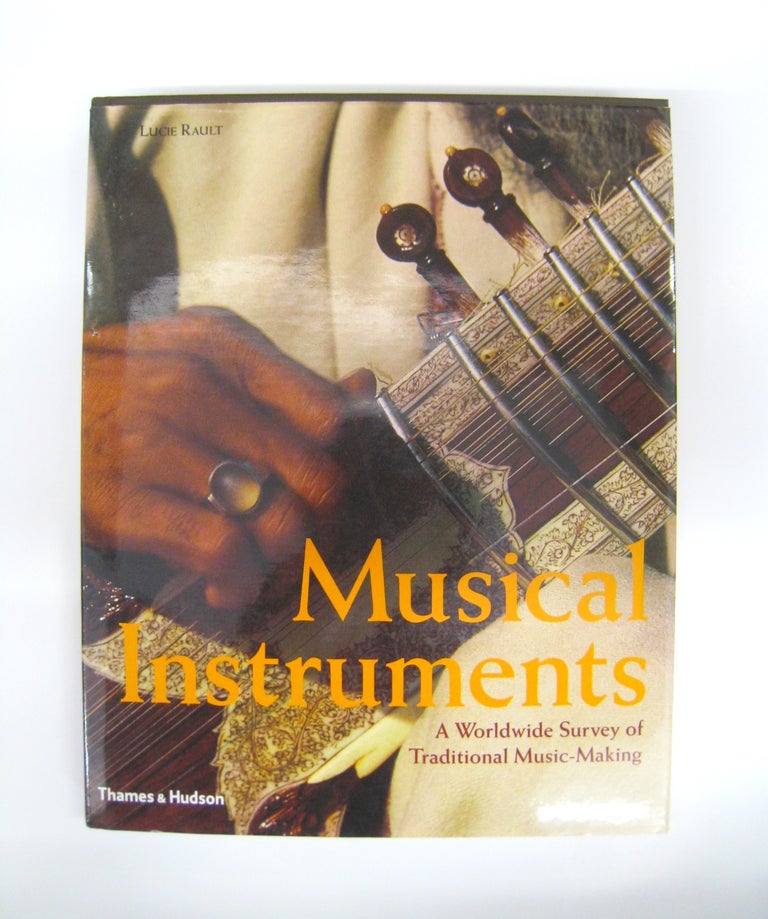This is a detailed cover image of a book titled "Musical Instruments: A Worldwide Survey of Traditional Music-Making." The top left corner features the name "Lucy Rault" in black text. Dominating the entire cover is a close-up photograph of the neck of a guitar, or possibly another cultural string instrument with intricate detailing on the neck and tuning pegs. A person's hand with a dark complexion, adorned with a large, round translucent ring on their ring finger, is prominently resting on the neck of the instrument. The individual appears to be wearing a white jacket. Towards the bottom of the cover, in large yellow text, the title "Musical Instruments" is displayed, followed by the subtitle "A Worldwide Survey of Traditional Music-Making" in smaller brown text. In the lower right corner, the publisher's name, "Thames and Hudson," is printed in small white text.